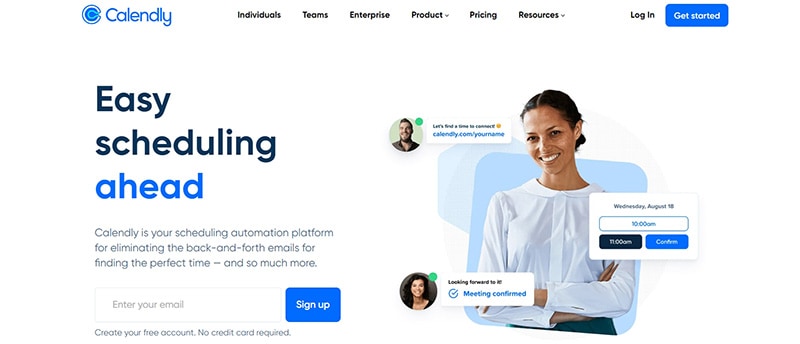This image is a screenshot from the Calendly website, a software tool designed to assist with online scheduling. The webpage features a clean, white background, including the header on the left side. The logo, displayed prominently, consists of the word "Calendly" written in a sans-serif font. To the left of the text, there is an elegant, stylized 'C' that resembles a circle, rendered in blue.

At the top of the page, the navigation menu, in a black font, lists options from left to right: Individuals, Teams, Enterprise, Product, Pricing, and Resources. On the far right corner, there is a Login option. Adjacent to this is a blue rectangle with white text that reads "Get Started."

The main section of the webpage features a headline on the left side in dark blue font that says "Easy Scheduling." Below this, in gray font, it explains, "Calendly is your scheduling automation platform for eliminating the back-and-forth emails for finding the perfect time and so much more." Beneath this text, there is an input field labeled "Enter Your Email," alongside a blue button with white text that says "Sign Up."

On the right side of the page, there is a photo of a smiling woman, seen from the waist up, who appears to be in her mid-20s. She has a light tan complexion, short dark brown hair, and is wearing a white blouse with her arms folded, suggesting a professional demeanor. To the right of her image, two smaller photos are displayed, likely serving as testimonials. The top photo features a white man with dark hair, while the bottom photo shows a white woman with dark brown hair.